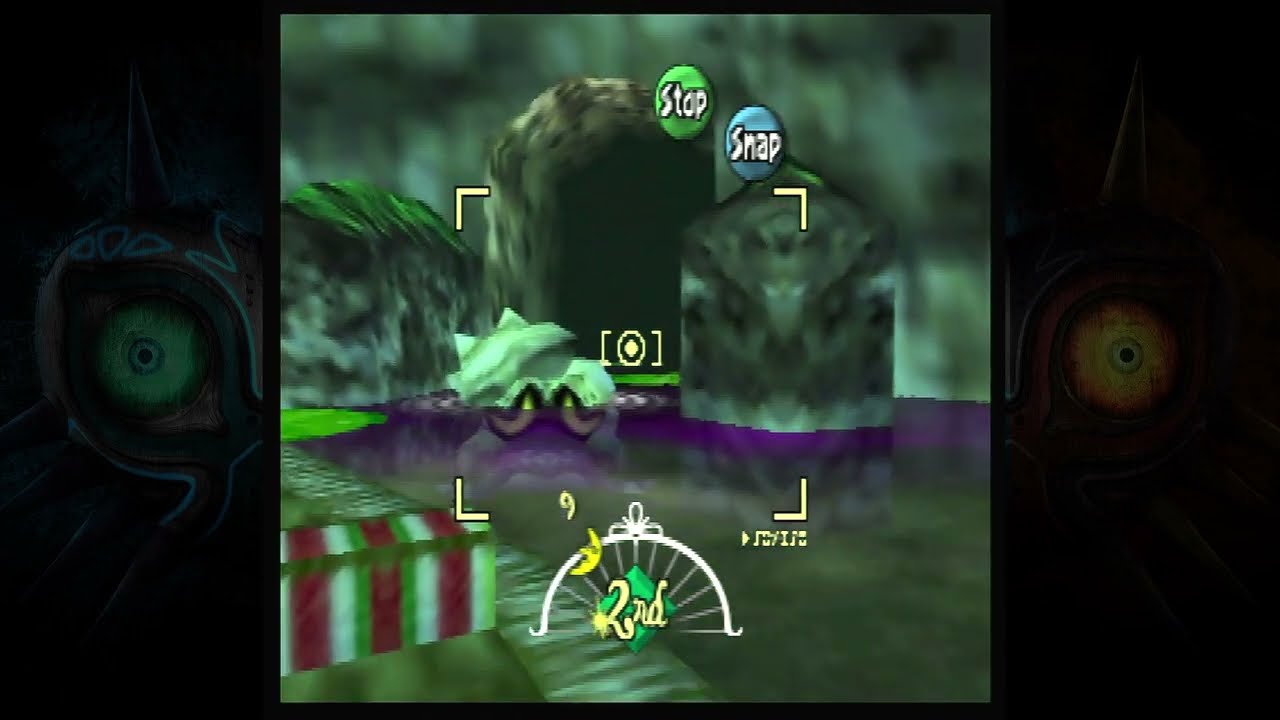The image is a colorful depiction from a children's video game, featuring a central scene and intricate details along its borders. The horizontal rectangular box has thick dark borders on both the left and right sides, each adorned with unique eyeball illustrations. The left border hosts an eye with a green sphere, a small blue circle, and a black dot at its center, surrounded by a casing with a spike on top and tentacle-like extensions at the bottom. Similarly, the right border features an eye with a yellow sphere and a black dot, encased with a spike on top and tentacle-like extensions moving to the right.

The main middle section of the image is somewhat blurry, resembling an entrance to a cave flanked by boulders. In front of the cave, there is a green vehicle approaching the entrance, carrying a round, lit green square. Above the cave entrance, a green circle inscribed with the word "stop" and a blue circle with the word "snap" indicate interactive elements. Below these signs, the foreground shows a blurry path leading from the bottom center toward the left edge of the image.

Additionally, at the bottom left, there's a half-opened box with vertical red stripes. Scattered throughout the scene, there are purple rocks and water, and a green creature with a sad face indicative of a video game character in distress. At the bottom of the screen, “second” is displayed in yellow lettering next to a green diamond, framed by white half-wheel spokes, further adding to the game's vibrant, animated style.